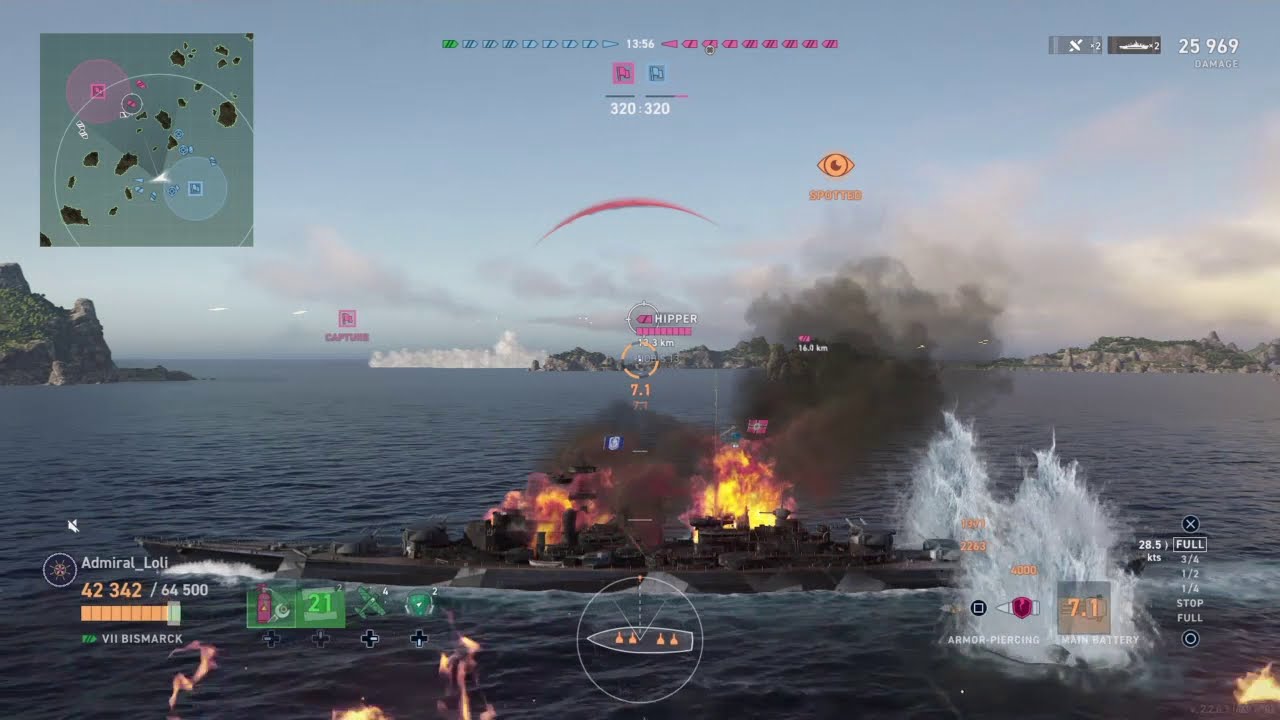The screenshot depicts an intense moment from the video game "World of Warships." In the foreground, a burning battleship appears to have just been struck by a torpedo or missile, with water splashing violently beside it. The top left of the screen features a mini-map showing the playfield, indicating the positions of various naval vessels, including battleships, aircraft carriers, and other ships from two opposing teams. Different indicators provide detailed information: the ship's damage status (42,342 out of 64,500 health), weaponry options (missiles, torpedoes, cannons), and the match time (13 minutes and 56 seconds). On the bottom left, the username "Admiral_Loli" is visible, while the top right and bottom right corners of the screen display additional statistics and indicators. The background illustrates a vast expanse of ocean, with an island and the mouth of a bay in the distance, highlighting the strategic elements of the game's environment. Flames and smoke dominate the scene, emphasizing the chaos and intensity of the battle, where the objective is to outlast the enemy team and emerge victorious.